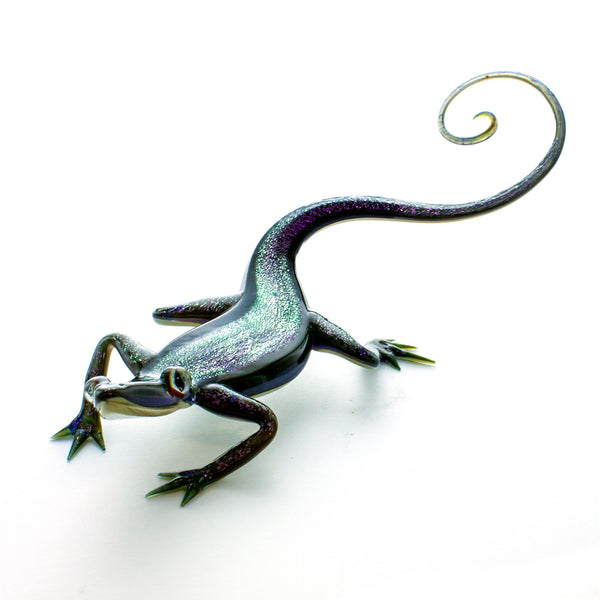In the image, there is a lifelike, multi-colored ceramic statue of a lizard, primarily rendered in various shades of green. The statue features intricate detailing: a back that transitions from light green adorned with gold flakes and speckles, shifting to darker green on the sides, and ending with a tan underside. The lizard's body is remarkably textured, highlighted by a light sheen as if reflecting light. It is positioned on a plain white background, and a shadow is cast beneath it, suggesting a flat surface. 

The statue depicts the lizard with a long, thin tail that gracefully curls upwards into a curlicue. It has four legs, though only three claws are visible, with the fourth obscured by its body. The front claws have three pointed claws, while the rear claws feature four sharp toes. The lizard's eyes are gold with black irises, giving it a beady, frog-like appearance as they bulge slightly from the sides of its head. Its gaze is directed to the left. The meticulous design captures the essence of a real lizard, making it a striking decorative piece suitable for a setting like a coffee table.